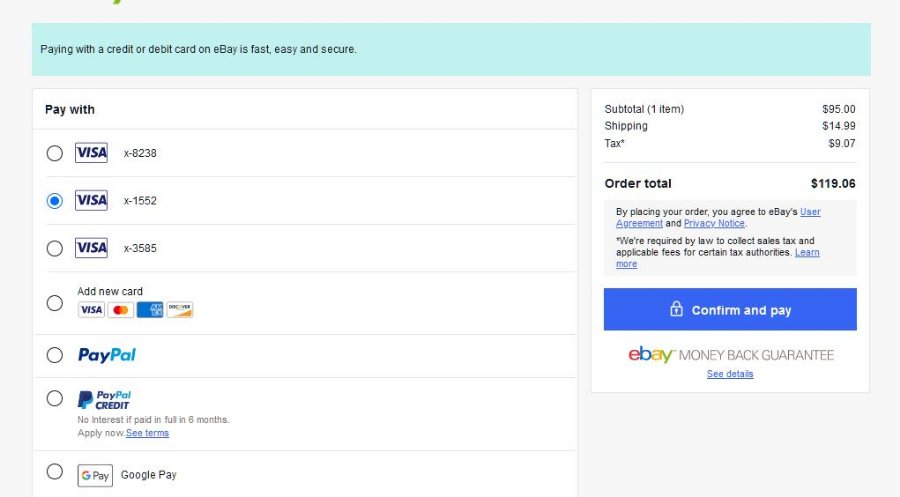The image showcases a payment selection interface on eBay. At the top of the screen, a teal-colored box prominently displays a message that reads, "Paying with a credit or debit card on eBay is fast, easy, and secure." Just below this, there is a list of available payment methods:

- Visa ending in 0238
- Visa ending in 1552 (selected, indicated by a blue highlight)
- Visa ending in 3585

Additionally, there is an option to "Add new card," and icons for Visa, MasterCard, American Express, and Discover are prominently displayed.

Further down, alternative payment methods are presented, such as "PayPal" and "PayPal Credit," with the latter offering a no-interest plan for six months for those who apply. "Google Pay" is also available as a payment option.

To the right of these options, a white square provides the order summary, including:

- Subtotal for one item: $95.00
- Shipping: $14.99
- Tax: $9.07

A line separates these details from the final order total, which is $119.06. At the bottom of this section, a prominent button labeled "Confirm and pay" encourages the user to finalize their purchase. An eBay Money-Back Guarantee is mentioned as a form of buyer protection at the bottom of the interface.